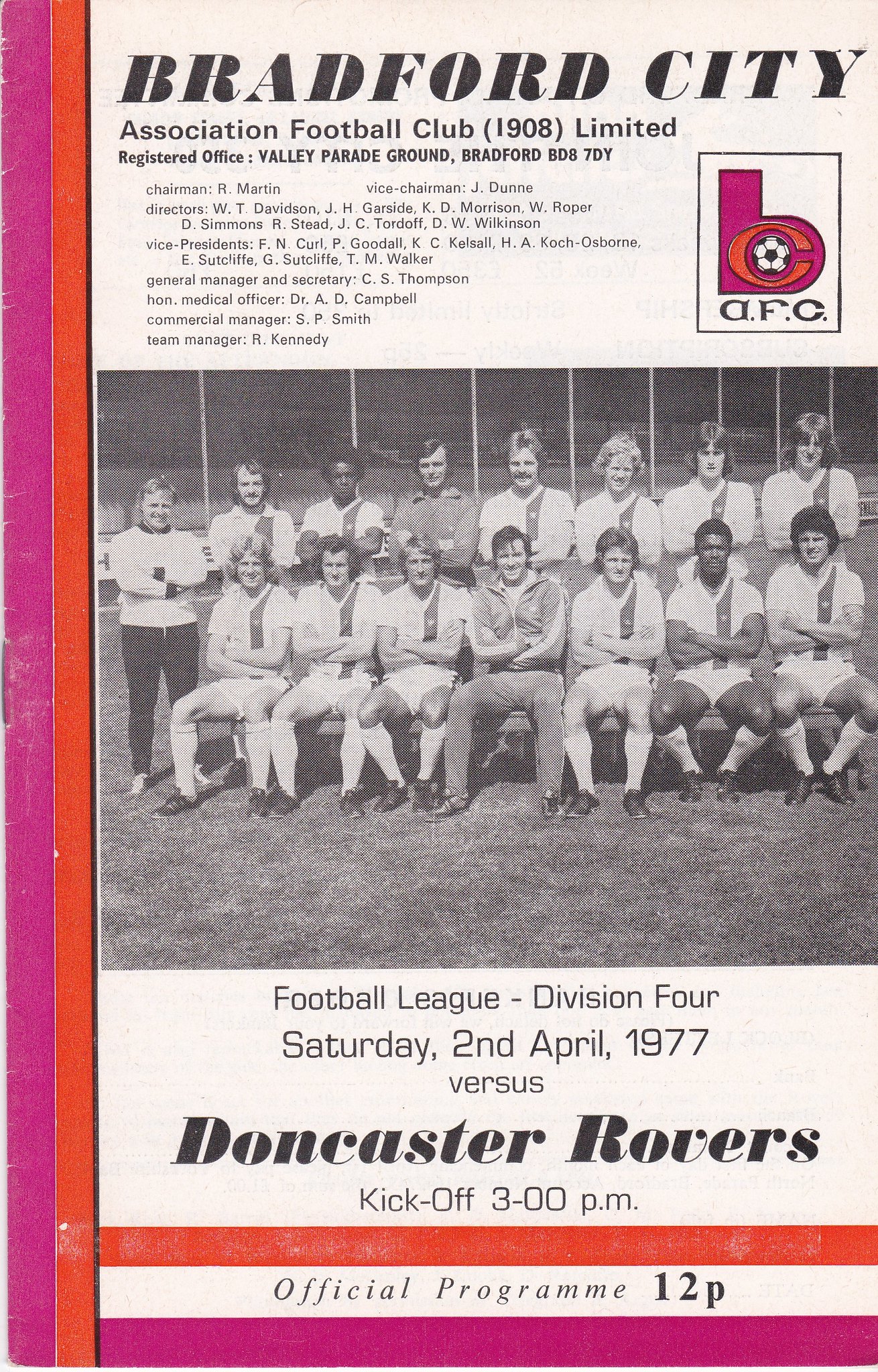The image is a scan of a football program cover mostly featuring a white background with accents. There are purple and orange borders along the left side and the bottom. At the top, bold italic black text reads "Bradford City," followed by "Association Football Club 1908 Limited," and "Registered office Valley Parade Ground Bradford B087DY." Below this are names and positions of the team management, including the Chairman B. Martin, displayed in a notably smaller font size. To the right, there is a logo featuring a pink letter 'B' with a red 'C' inside and a soccer ball at the center, accompanied by the text "A.F.C." beneath it.

Centrally positioned is a black and white photograph of the football team. The team comprises two rows: the front row, seated, has seven players with one coach in the middle not wearing a jersey, and the back row, standing, has eight players, including an assistant coach. Notably, most players are white, with two black players identified as the second from the right in the front row and the third from the left in the back row.

Underneath the image, black text announces the match details: "Football League Division 4, Saturday, 2nd April 1977, versus Doncaster Rovers, kickoff 3 p.m." This is followed by the designation "Official Program 12P." The program is additionally decorated with a red stripe and a pink stripe encapsulating the words "Official Program 12P," which are also mirrored along the left edge.